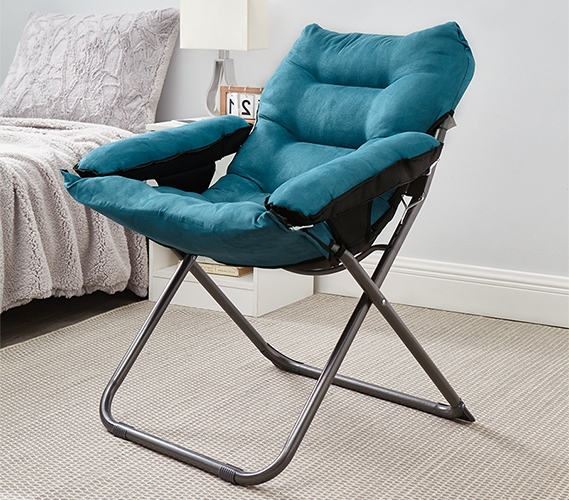This image features a teal, foldable chair with cushioned back and padded arms, set awkwardly within a bedroom. The chair, which typically belongs in an outdoor setting, contrasts sharply with the room's décor. Resting on an ivory Berber carpet, the chair's metal frame creates a stark juxtaposition against the soft furnishings. The room includes a twin bed with an off-white, fuzzy blanket and a matching pillow. A nightstand beside the bed hosts a modern white lamp, a calendar displaying "12," and an open lower shelf holding books. The walls are adorned with wainscot molding and painted a very light gray, harmonizing with the overall subdued and cozy bedroom aesthetic, which makes the chair's presence feel even more out of place.